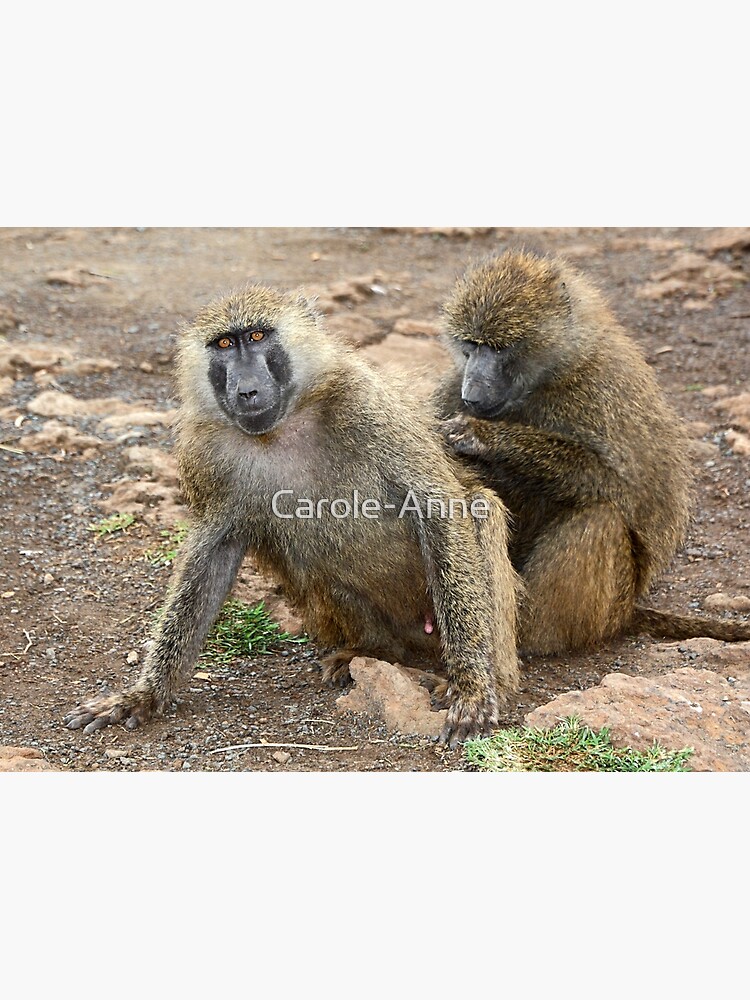In a vertically aligned rectangular image, framed by thick light gray borders at the top and bottom, a horizontal picture showcases two medium-sized primates in a natural setting of dirt, loose rocks, and sparse grassy patches. The foreground monkey, with striking gold eyes and a black and gray mouth and snout area, gazes directly at the camera. Its face is framed by some white fur, while the rest of its body is covered in spiky brown fur with varying shades of tan and brown. This monkey leans forward, its arms planted wide on the ground. 

Behind it, a second monkey appears to be grooming the first, focused intently on its task or the back of the front monkey. This background primate has a darker brown coat, lighter fur around the sides of its head, and a partially visible black face. Both monkeys sit on a mostly barren patch of land, with some green grass and leaves scattered amidst the predominantly tan and brown terrain. Across the center of the image, the name "Carol-Anne" is prominently displayed in white print, serving as a watermark.